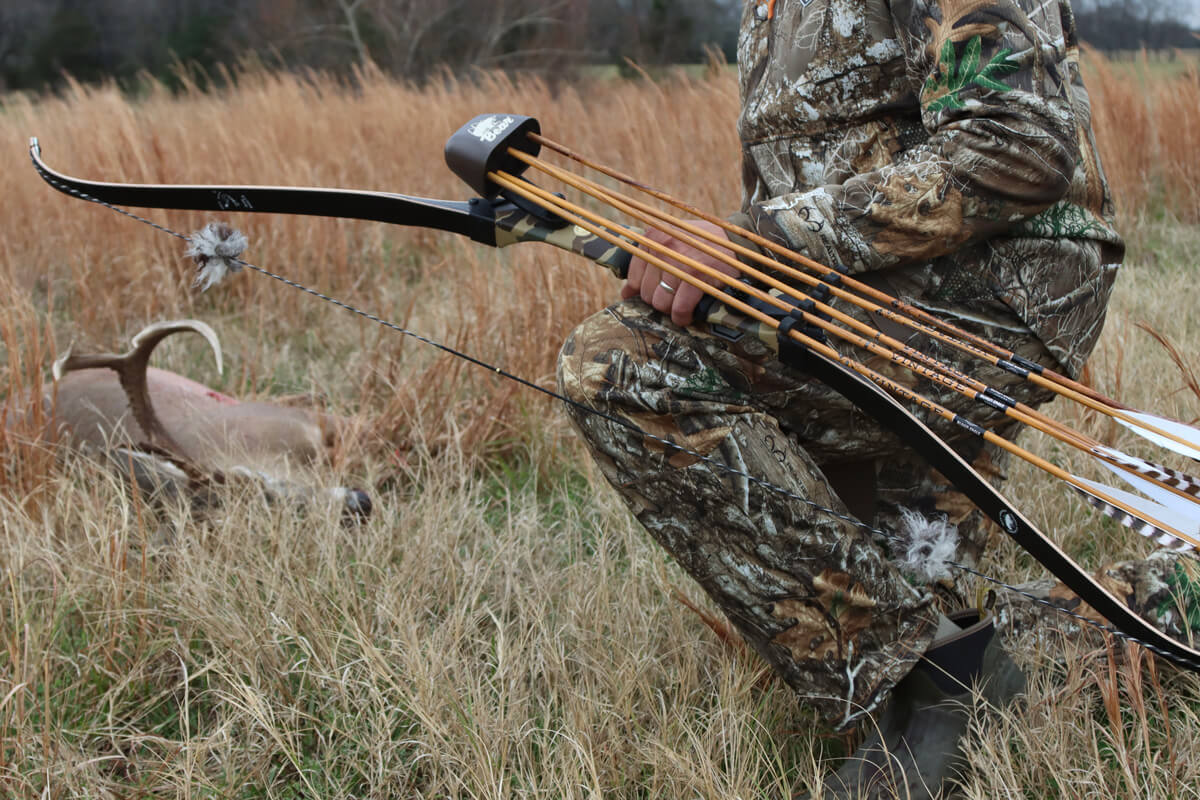A kneeling hunter, dressed in a full camouflage outfit with patterns resembling branches and leaves, is captured in a grassy field surrounded by tall weeds. His attire includes a camo shirt and pants, a wedding ring, and distinctive flat, fluffy-textured hiking shoes. In his left hand, he holds a professional black bow with a green and black camouflage handle. The bow is equipped with an arrow holder containing five arrows, each adorned with white feathers marked by gray stripes. On the ground, a few feet away and partially concealed by the tall grass, lies a deer with large horns and a visible bloodstain near its heart, indicating where the arrow struck. The background subtly shows an expanse of trees, adding depth to the outdoor setting.